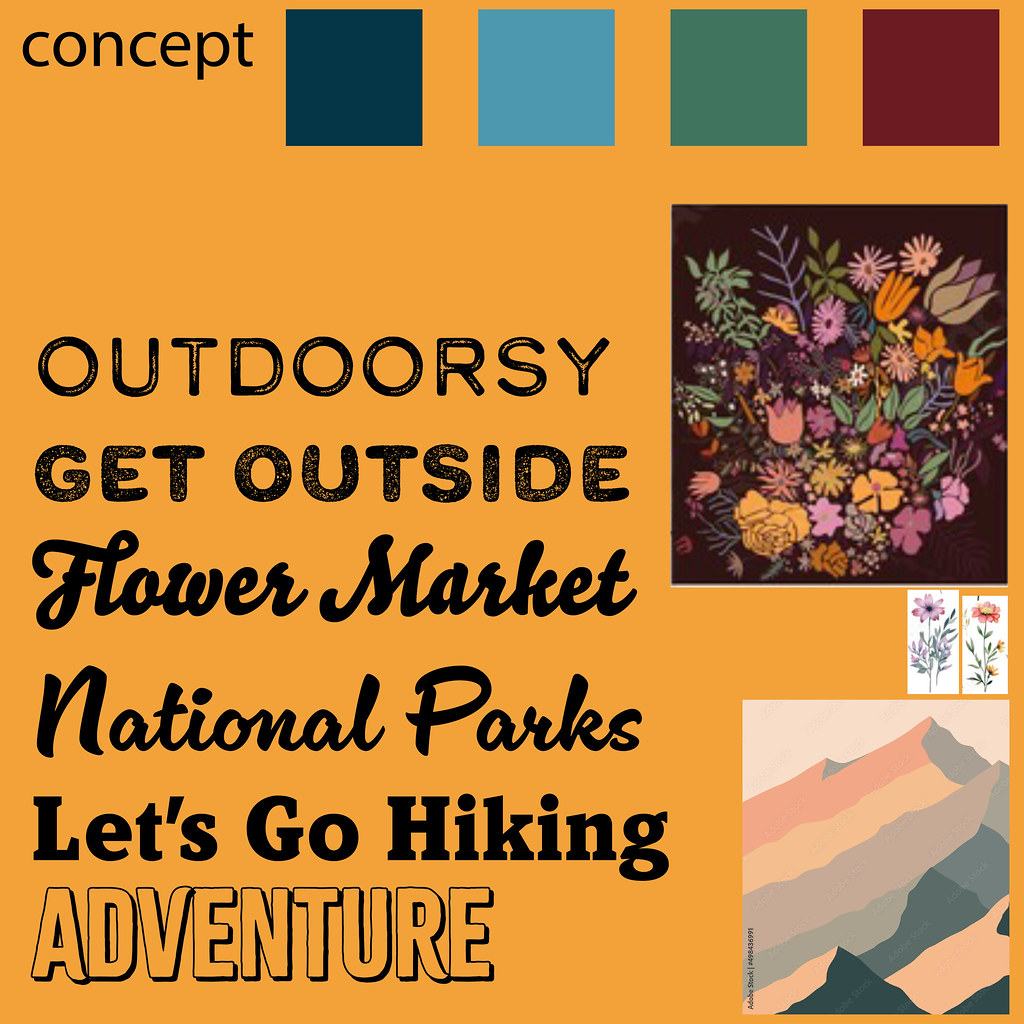This image features an orangey-tan background and resembles a card layout. In the top left corner, the word "Concept" is prominently displayed. Adjacent to this, four colored squares appear—dark blue, light blue, sage green, and maroon red. On the left side of the card, slightly above the middle, there are five lines of text in various sizes and styles: "Outdoorsy," "Get Outside," "Flower Market" (in cursive), "National Parks," "Let's Go Hiking," and "Adventure" (in large, outlined capital letters). 

To the right of the colored squares, a black-bordered photograph showcases a vibrant bouquet of flowers in colors like purple, blue, green, orange, and yellow. Beneath this photograph, two smaller white rectangles feature individual flowers. The bottom right corner contains a sketch of a mountain range, rendered in shades of tan, yellow, gray, and black. The array of colors throughout the image includes orange, black, dark blue, light blue, sage green, dark red, purple, pink, and tan, creating a visually rich and detailed composition.